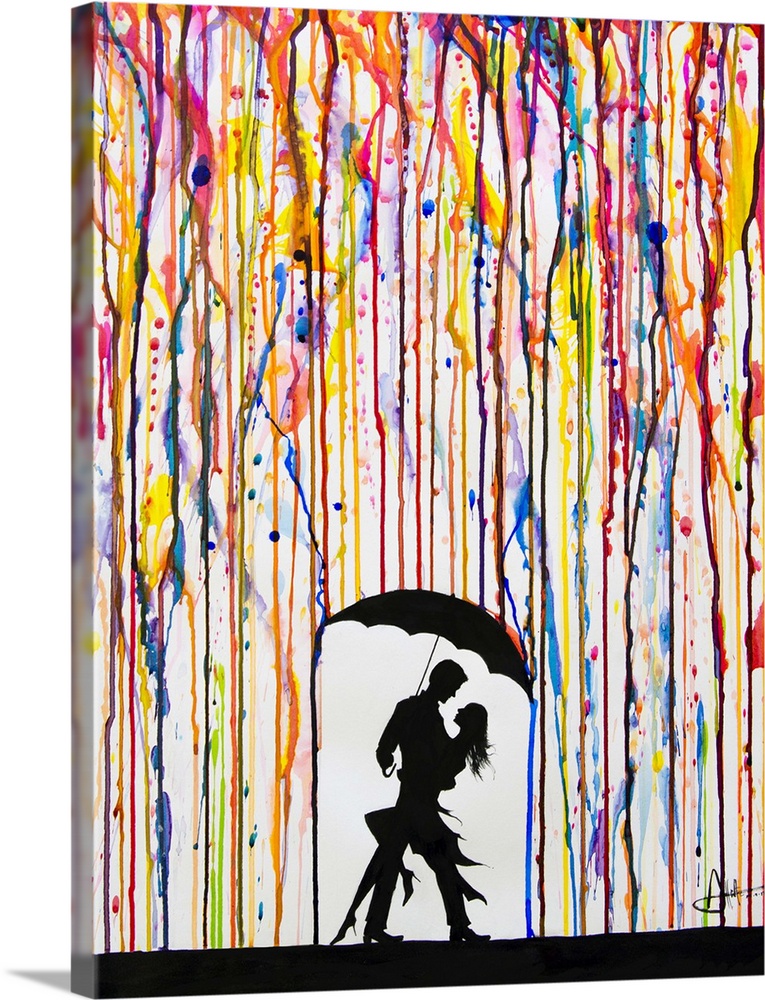In this vertically aligned rectangular painting, we see an intriguing and colorful piece set against a white canvas, giving it a 3D effect with visible edges on the left side. The canvas is adorned with an array of vertical streaks and splotches representing the colors of the rainbow—blue, yellow, green, red, pink, and orange—creating a vibrant yet somewhat chaotic background that is thicker at the top and thins out towards the bottom. These streaks and dripping paint seem to bleed into one another, generating overlapping hues and additional colored dots throughout the image. 

The focal point of the painting is positioned at the bottom center, where a solid white archway devoid of colorful streaks highlights a black silhouette of a couple. The man, dressed in a suit, holds the woman, who is in a dress and high heels, as they dance together under an umbrella. The umbrella, also entirely black, creates a stark contrast against the white background beneath it, symbolically catching the rain of colors dripping from above. The very bottom of the painting features a thick, solid black strip running horizontally across the width of the canvas, adding a grounding element to the scene.

Additionally, there is a signature in black located in the lower right corner of the canvas, although it is unreadable. A shadow cast at the bottom left corner further enhances the painting's dimensionality, completing the visual narrative of this captivating artwork.